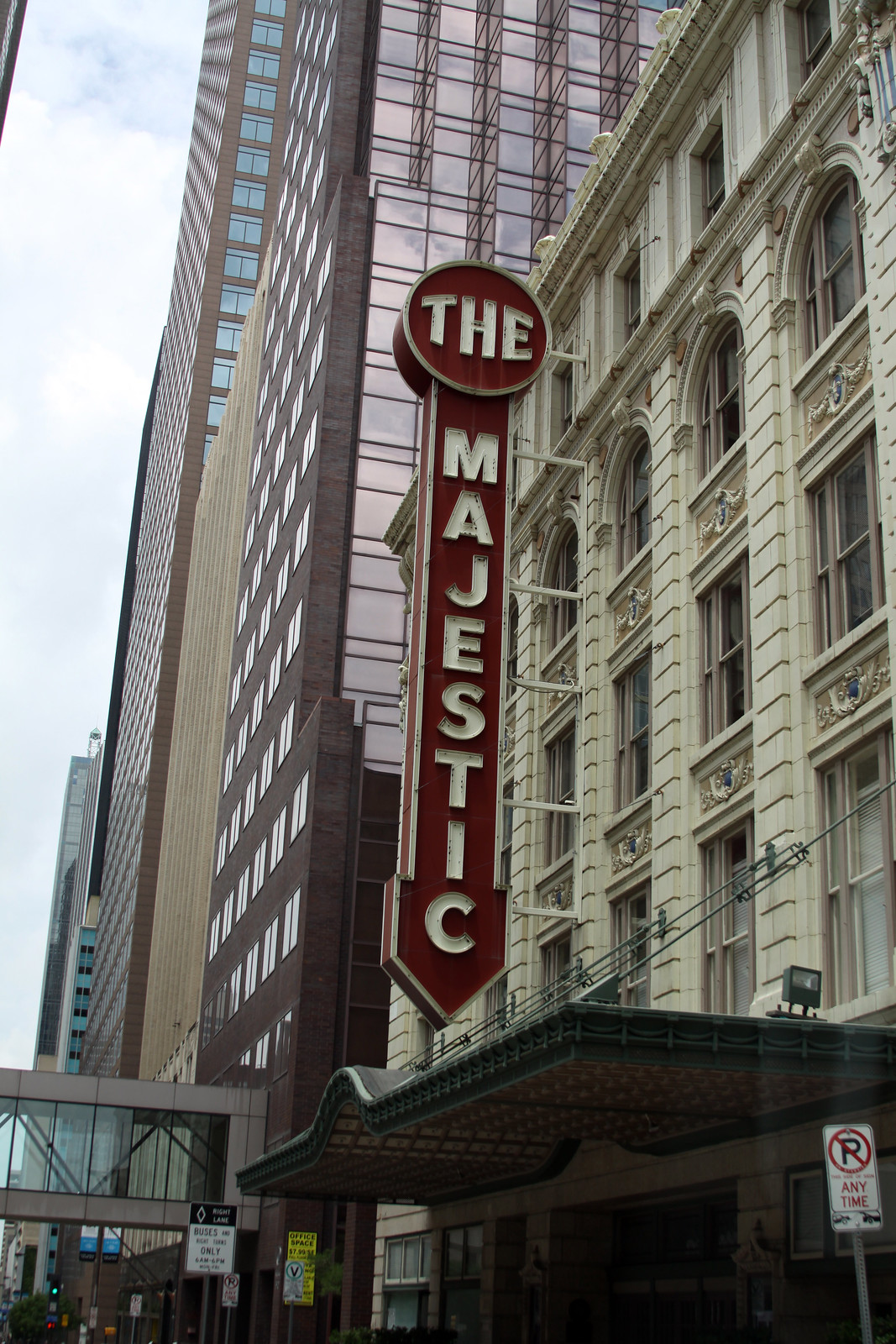The image captures the side of a city building, with a camera angle slightly pointed upwards from street level. The nearest building in the frame is a structure of about ten stories or fewer, featuring a prominent, old sign jutting out from the wall. This sign, bordered by neon lights, bears the words "The Majestic" in white letters. The sign's design includes a round circle around the text with an additional circle pointing toward what appears to be an entrance. Below the sign is a green metal overhang with a light affixed to its side, and a street corner sign that reads "No Parking Anytime."

In the backdrop, towering skyscrapers with extensive window-covered facades stretch high into the sky, dwarfing the nearby buildings. The sky visible in the image, located toward the left edge, is largely overcast, suggesting a cloudy day. Additionally, there is an overhead walking bridge connecting two of the larger office buildings in the distance. This intricate composition highlights the blend of historical and modern architectural elements within the urban landscape.